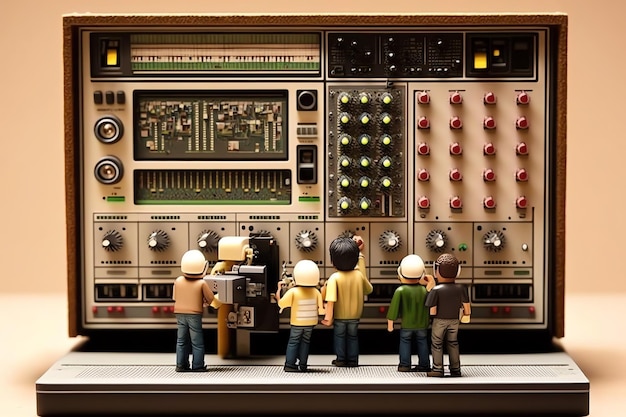The image is a digitally created artwork featuring a mixing console styled to appear like a large amplifier or radio in a landscape orientation. The console, a horizontal rectangular box, is detailed with a green and white window on the top left, numerous dials and knobs beneath it, and sections with exposed circuitry. The right side features two vertical panels with multiple jack connections. Below these elements, there is a row of ten silver knobs with black text underneath. Standing on a wide, shallow platform in front of the console are seven miniature construction worker figures. These tiny engineers, wearing white hard hats and protective vests, are facing away from the viewer and appear to be examining or operating the console. The detailed setup, combining realistic elements with digital art, creates the illusion of tiny workers interacting with a vast, complex piece of audio equipment.